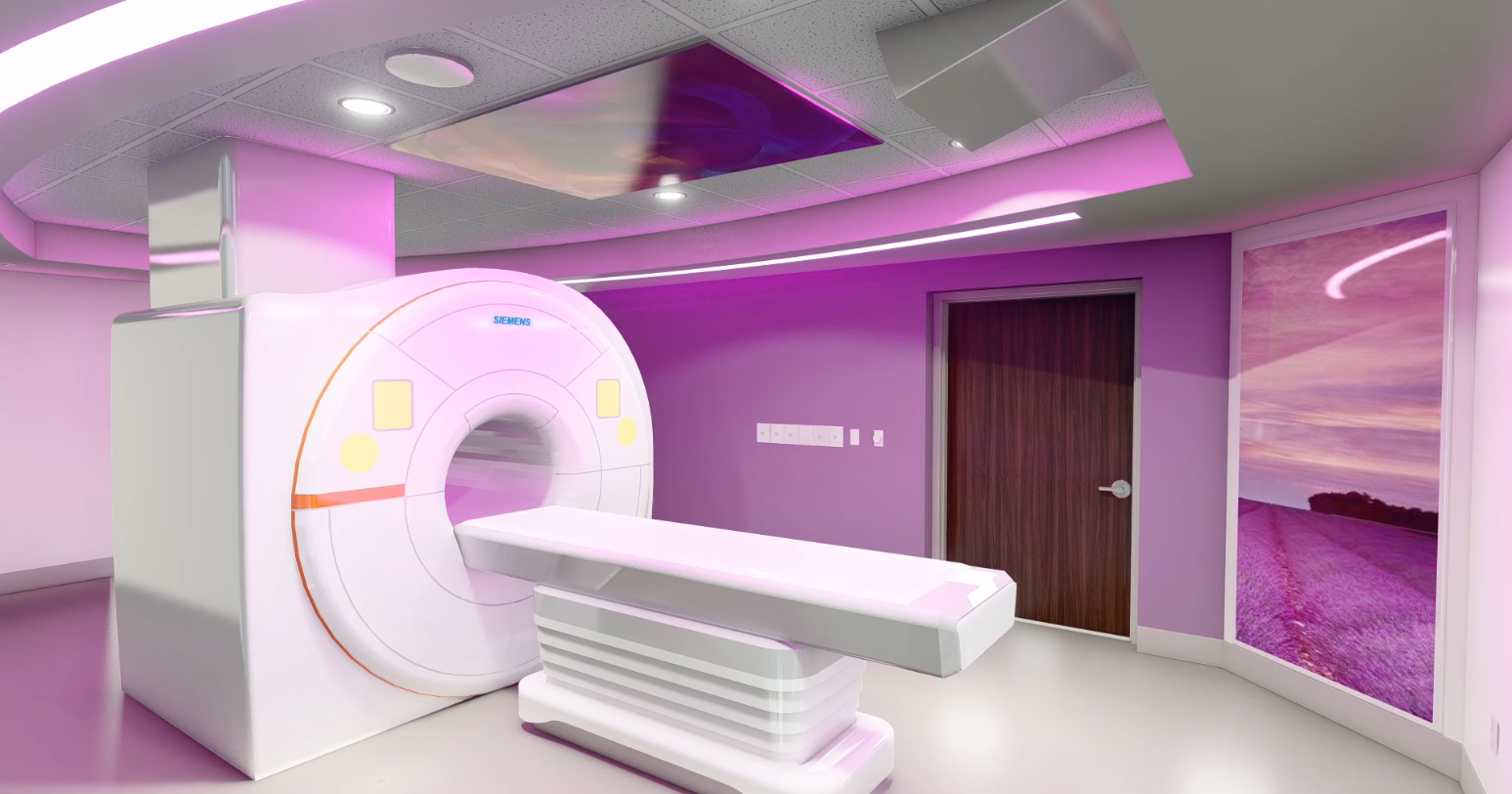The photograph captures a modern and pristine medical imaging room, likely part of a hospital or radiology lab. Dominating the center of the room is a white MRI scanning machine branded with the word "Simons" in blue letters. The machine features a large, circular opening with a smooth, sliding platform designed for patient alignment. The walls are a striking purple color, creating a soothing and calming ambiance, complemented by a shiny, light grey floor. Overhead, the grey ceiling is equipped with circular-shaped lights providing ample illumination. A large, brown wooden door is situated on the front wall, suggesting an entry or exit point. The overall setting appears new and meticulously maintained, with a tranquil and orderly atmosphere.